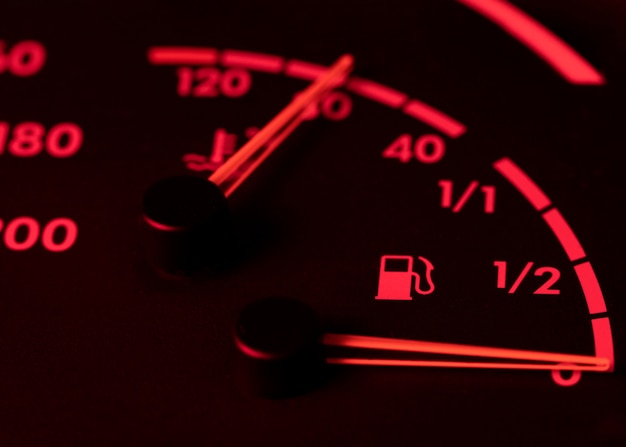This image is a detailed close-up of a car's dashboard, prominently featuring the speedometer and fuel gauge. The dashboard has a dark, black background with bright red indicators and numbers, creating a striking contrast. On the left side, the speedometer needle points to 80, with markings ranging from 40 up to 120. To the right, the fuel gauge, shaped like a semicircle, displays readings from 1/1 (full) to 1/2 and then to 0 (empty); currently, the needle is at 0, indicating an empty tank. The design suggests the car's internal lights are on, illuminating the gauges in vivid red and highlighting critical information like the oil level marker and the fuel indicator. The elaborate red lighting indicates that the vehicle's ignition might be off.